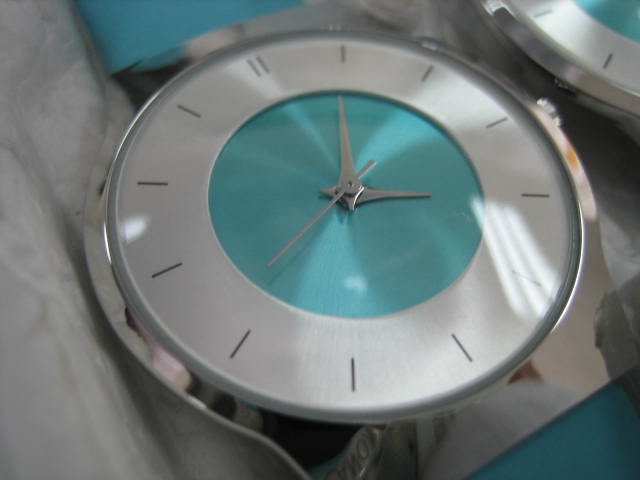The image showcases an ultra-close shot of a sleek, modern watch. Encased in a gleaming silver frame and protected by a glass covering, the watch features a polished silver crown used for time adjustment. The timepiece is distinguished by its vibrant aqua blue band, imparting a stylish and contemporary flair. At the center of the watch face, three silver hands—each meticulously designed—indicate the time: a long, slender second hand, a pointed minute hand, and a shorter, equally pointed hour hand. The watch face itself is adorned with minimalist hour markers, with the positions 1 through 12 identified by simple numeric indices, except for the 12-o'clock position which is denoted by double slashes. The watch has been thoughtfully positioned against what appears to be a textured graphite or quartz surface, enhancing its sophisticated aesthetic.